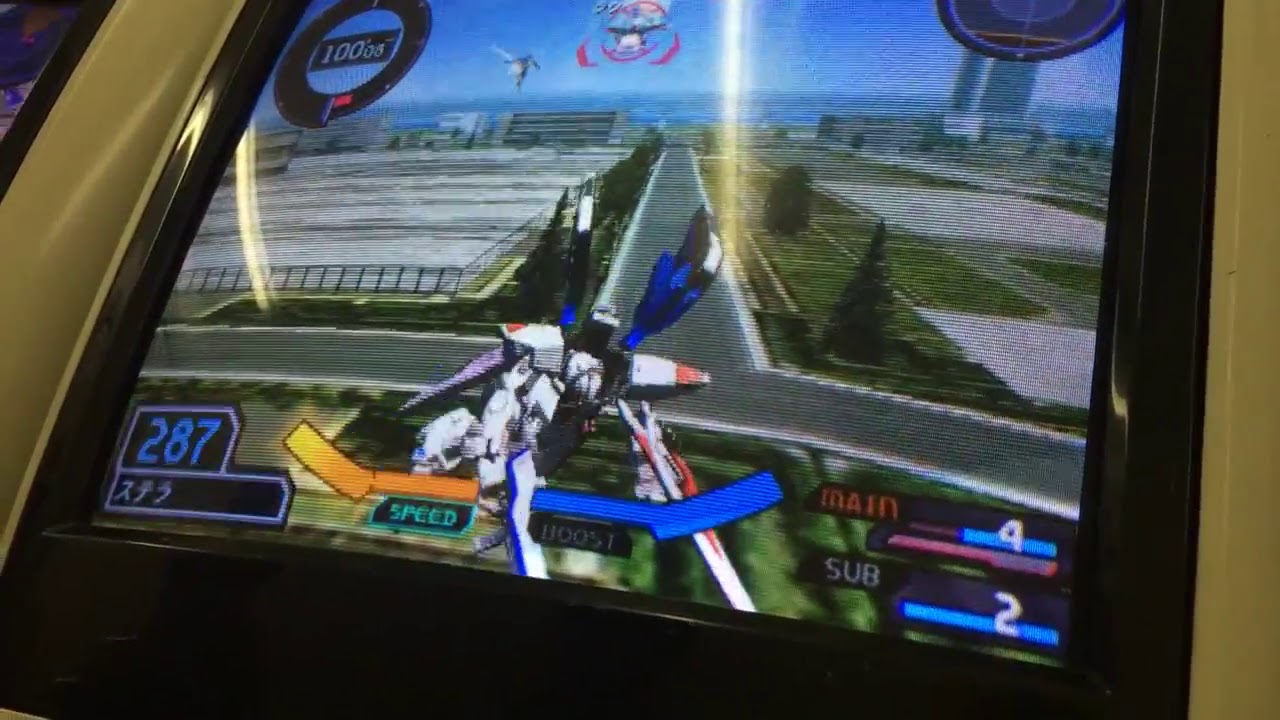The image captures a photograph of a screen from an original Gundam arcade game, taken at an offset angle. The screen shows a character mid-flight, targeting a distant figure, with several game indicators visible. On the bottom left, blue numbers display a score of 287, next to which an orange bar labeled "Speed" and a blue bar labeled "Boost" are visible. The right side of the screen features the word "Main" in red followed by the number 4 in white, and "Sub" with the number 2 in white. In the top left corner, there's a mileage gauge showing 100. The game's graphics have a lower video quality, reflective of its age, yet the surrounding plastic housing the screen, though slightly discolored, appears to be holding up well. The background portrays a scene with a blue sky, possibly the roof of a factory to the left, and a cityscape to the right. The ground below features blurry trees and white areas, with a glimpse of a distant building. The image does not include the player or the entire screen in full.